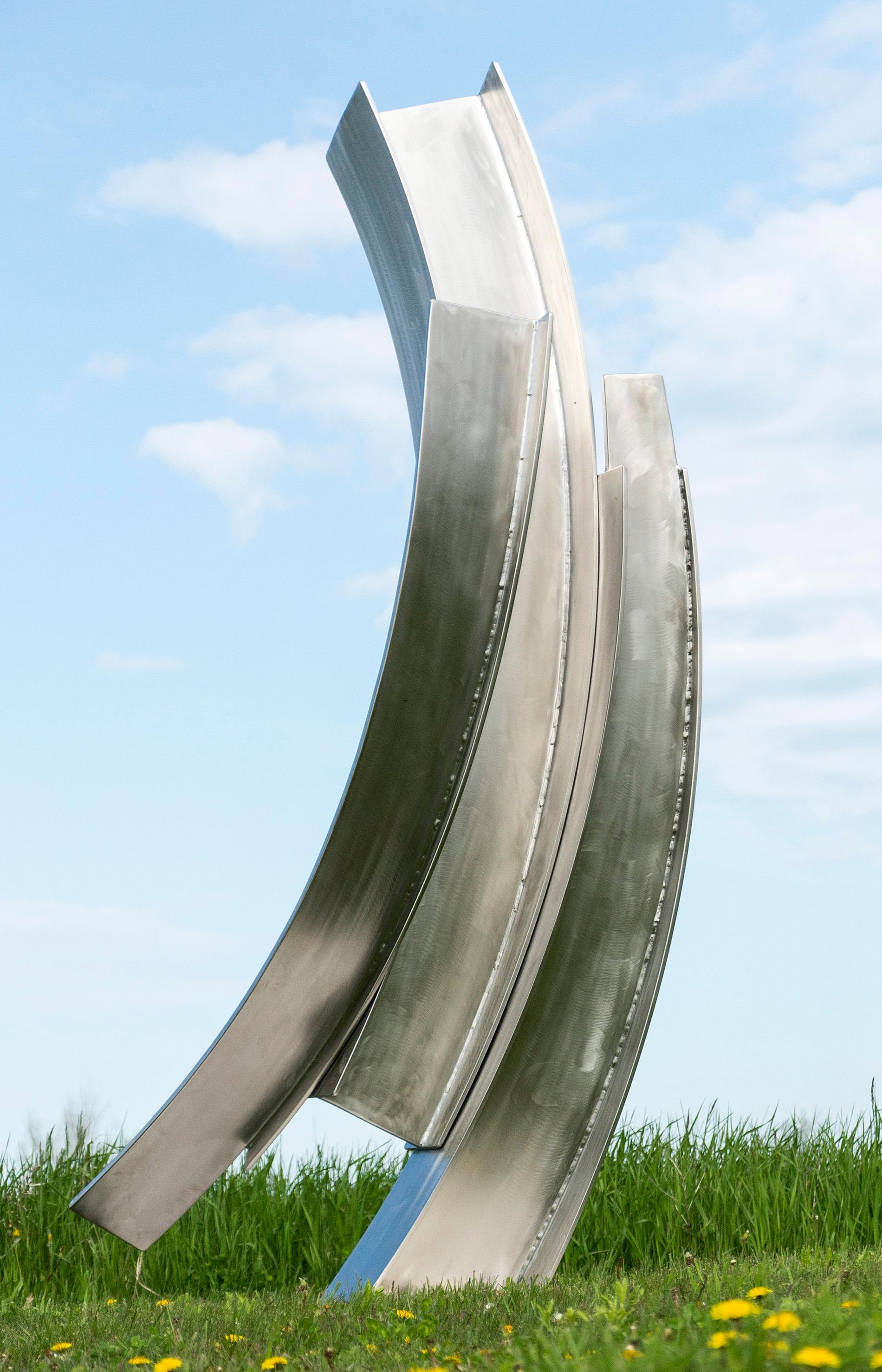This photograph captures a striking abstract outdoor sculpture in a grassy field. The sculpture, made of shiny silver metal, comprises three curved I-beams. The first piece originates from the ground, curving up and slightly to the left. The second piece, resembling a square flange post, curves similarly and connects to the first piece about halfway up. The third piece curves in front of the second, attached at the bottom and extending slightly lower than the middle piece.

The field in which the sculpture stands has shorter grass peppered with yellow dandelions, contrasting with taller, darker green grasses in the background. The sky above is a clear, light blue with a few wispy white clouds, particularly concentrated on the right side of the image. The vertical composition of the photograph emphasizes the height and elegance of the sculpture against the serene, natural backdrop.